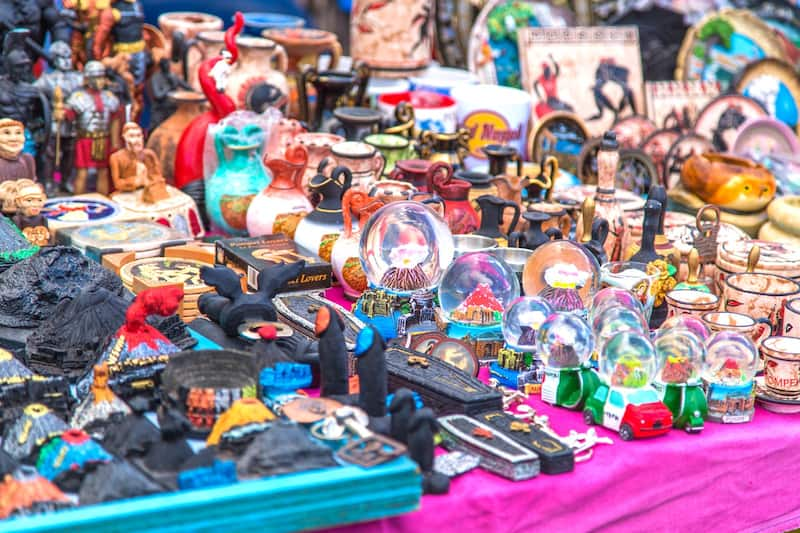The image depicts a bustling market table brimming with an eclectic array of souvenirs and knickknacks, set against a landscape orientation. The table is covered with a mix of pink and blue cloths and laden with various ceramic and decorative items. Central to the display are numerous snow globes, featuring unique designs such as miniature cars, coffee mugs, and Santa Claus heads encased within the globes. 

On the left-hand side of the table, there are small volcano-shaped models and distinctive black statues with painted tips. A collection of coasters and several small sculptures, including ones resembling Roman soldiers, can also be seen towards the back of the tableau, adding a historical touch. 

Moving towards the right, more snow globes appear, alongside intricately painted cars in green, white, and red, hinting at an Italian theme. Prominent among the items are numerous clay vases and tea cups, one of which prominently displays "Pompeii" in red letters, perhaps indicating the market's locale or theme. The rightmost section features additional plates and paintings, rounding out the vibrant assortment of souvenirs.